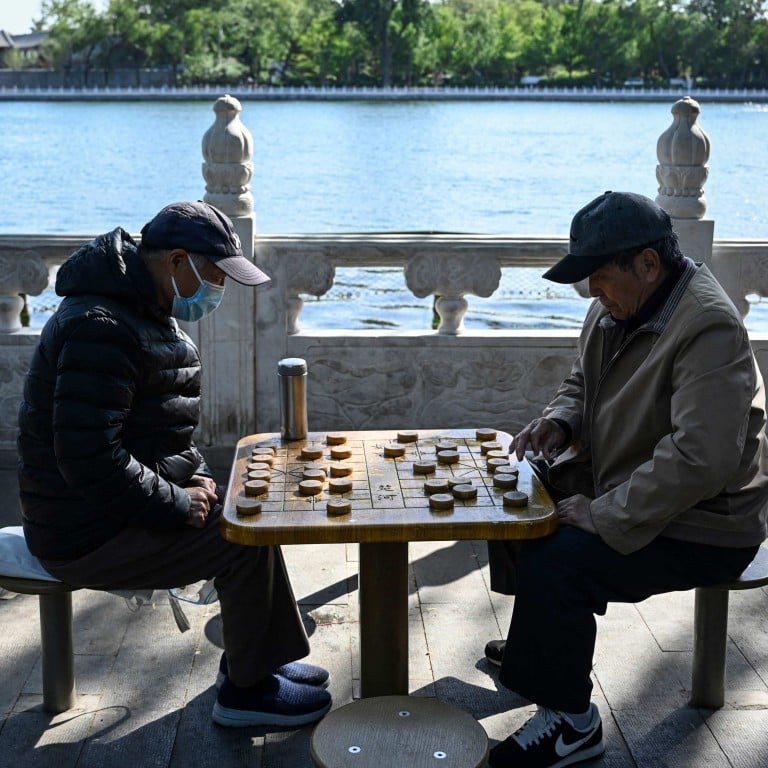Two elderly men are absorbed in an intense game of Chinese chess at a square wooden table built into the cement ground. Their seats, round stools mounted on metal posts, are also fixed into the sidewalk. The player on the left, wearing a blue face mask, a baseball cap, and a black puffy jacket, appears more concerned about COVID-19. The man on the right, dressed in a khaki jacket and a baseball cap, has visible wrinkles on his skin. The game involves moving large, round wooden pegs with symbols across a grid etched into the tabletop. A thermos sits on the far left side of the table. Behind them, a decorative stone or marble fence separates them from a shimmering blue lake, with lush green trees lining the opposite shore. Both men remain intensely focused on their game, oblivious to the camera capturing the scene.